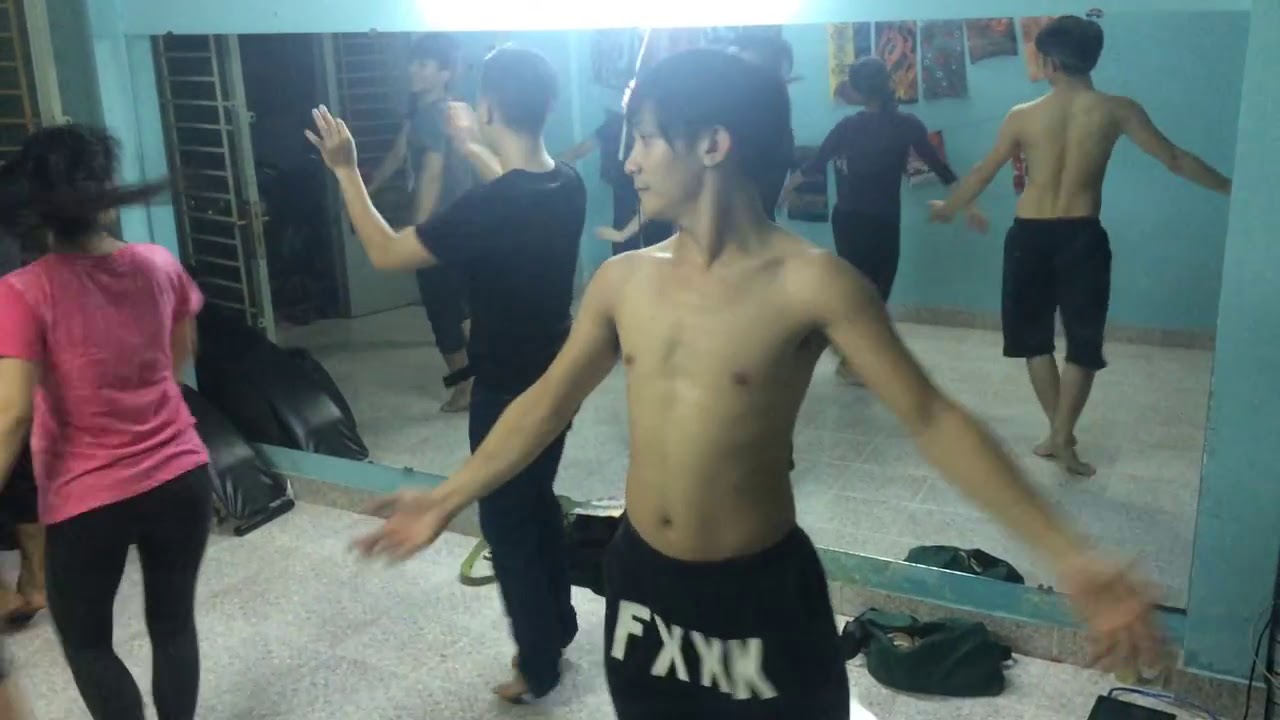In this indoor image set on a hard tile floor, we see a dynamic scene that appears to be a dance studio, possibly in the middle of the day. Central to the composition is a shirtless young man with medium-length hair looking to the left. His arms are splayed out at approximately 45-degree angles, with his palms facing outward, suggesting movement or a dance pose. He is dressed in black shorts with the bold text "FXXK" displayed on the front. 

To his left stands a female figure in a pink shirt and black pants; she seems to be looking slightly to the right or possibly walking away. Another male figure is positioned behind the shirtless man; he is clad in an all-black outfit with long pants and has his hands raised, palms up, as if pushing against the sky. Further left, a woman's reflection in a large mirror on the back wall reveals her wearing a dark brown shirt and black pants, mimicking the main pose of the shirtless man. Within the mirror, another young man in a gray shirt and black pants appears to be engaged similarly in some kind of dance form, with his arms down as if pushing against the ground.

Scattered on the floor are various bags and items, hinting at a casual and active environment. The overall scene is vibrant with colors like pink, black, tan, white, green, orange, and yellow subtly dispersed throughout, contributing to the bustling yet focused atmosphere of what seems to be a dance class or practice session.